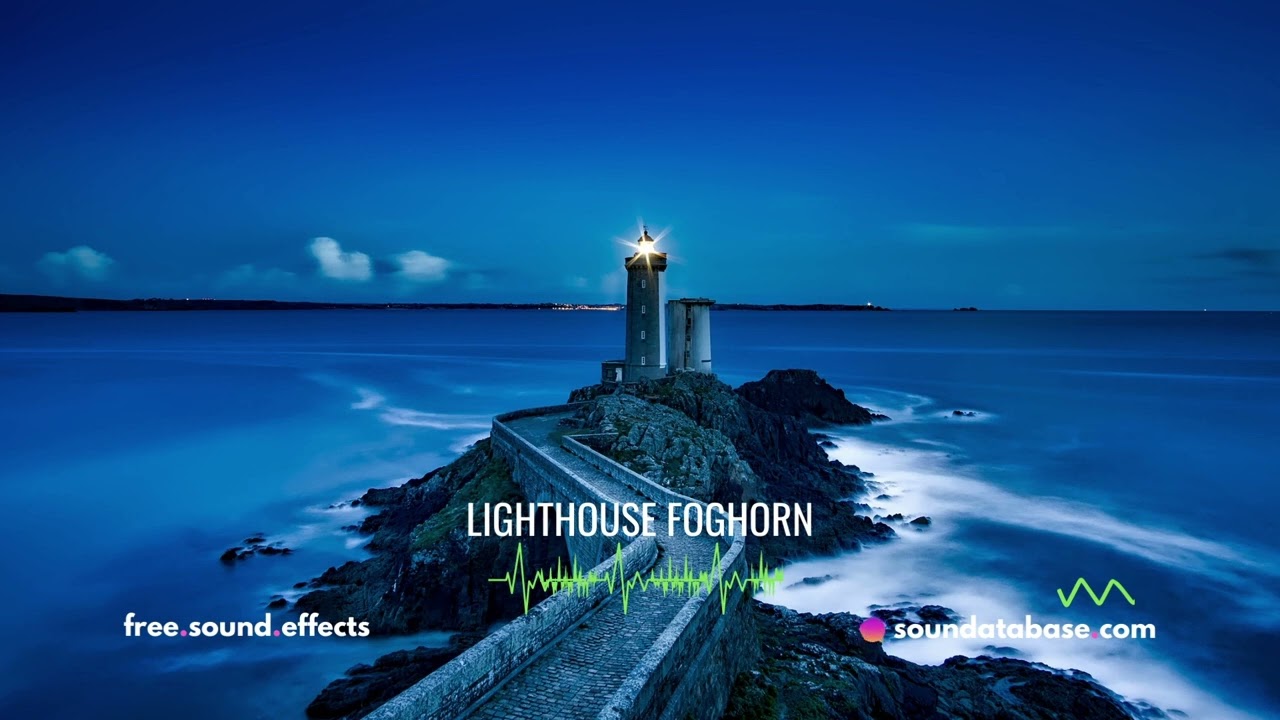This captivating advertisement photo showcases a picturesque nighttime scene of a lighthouse situated on a rugged rocky shore, dramatically illuminated under a cloudy sky. The lighthouse, standing tall with its four windows and an adjoining small silo, casts a bright yellow beam of light that pierces the night. A long cobblestone path leads up to the lighthouse, bordered by the ocean's crashing waves. In the far distance, a small town or city is faintly visible under the cloud-streaked sky, adding depth to the landscape. 

Central to the image, bold white text reads "Lighthouse Foghorn," accompanied by a green sound wave graphic below it. The lower left corner features the website "free.sound.fx" written in a combination of pink and white text, each word separated by small pink dots. On the lower right, "SoundDatabase.com" is displayed in white text, accented by a pink circle and a lime green sound wave bar partially overlaying the text.